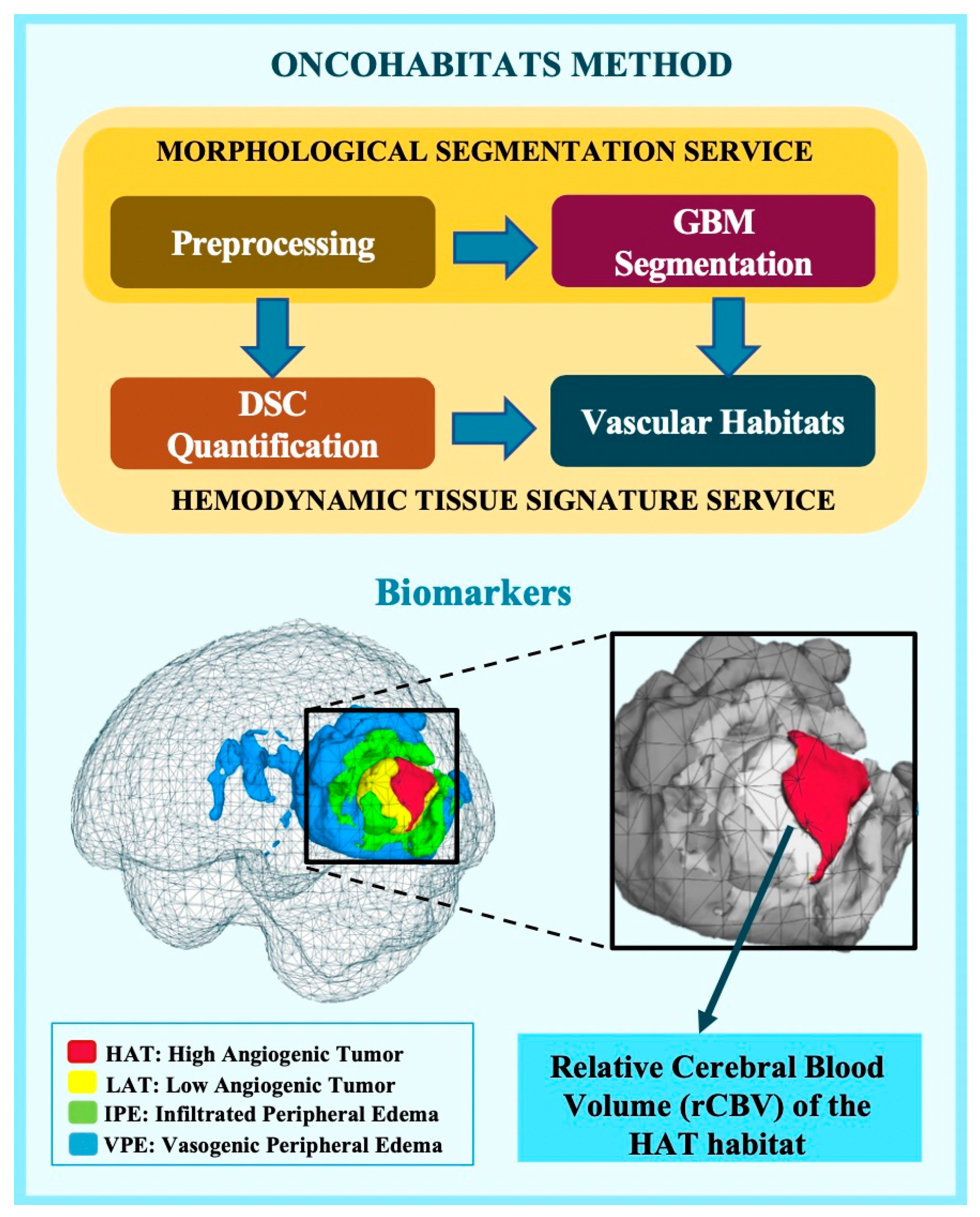The image depicts a detailed medical diagram on a pale aqua background, titled "Uncohabitous Method" at the top in blue lettering. It illustrates a flowchart with interconnected boxes highlighting processes such as "Preprocessing," "DSC Quantification," "GBM," "Segmentation," and "Vascular Habitus," culminating in the "Morphological Segmentation Service." Below the flowchart, the text reads "Hemodynamic Tissue Signature Surface" with the word "Biomarkers" in green. The diagram also includes a 3D scan of a brain, with a specific region highlighted in greens, blues, yellows, and reds, accompanied by a close-up labeled "Relative Cerebral Blood Volume of the Habitus." Four differently colored boxes (brown, red, orange, and blue) in the central section point toward various aspects of the segmentation service.